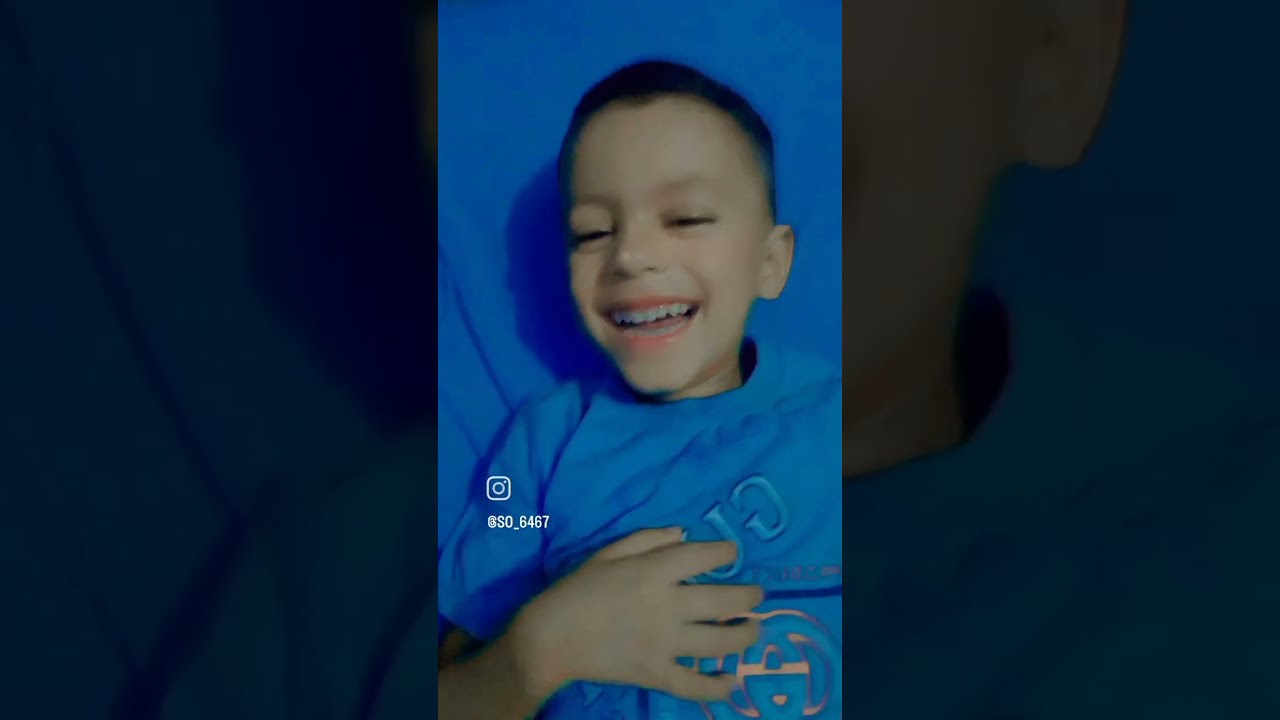This image captures a joyful boy, approximately seven or eight years old, with short black hair and light skin. He is lying down on a blue sheet that matches his blue short-sleeved shirt, which appears to have the letters "G" and "U," possibly indicating a Gucci logo. The boy is in the center of the horizontal rectangular picture, smiling widely with his teeth showing and his right arm bent and resting on his chest. The background and his shirt blend seamlessly into blue. On either side of the central image, there are blurred and darker close-ups of the boy, with the left showing part of the blue sheet and the right showing his cheek and ear, creating a focused effect on his happy expression. The image exudes a sense of delight and casual comfort.